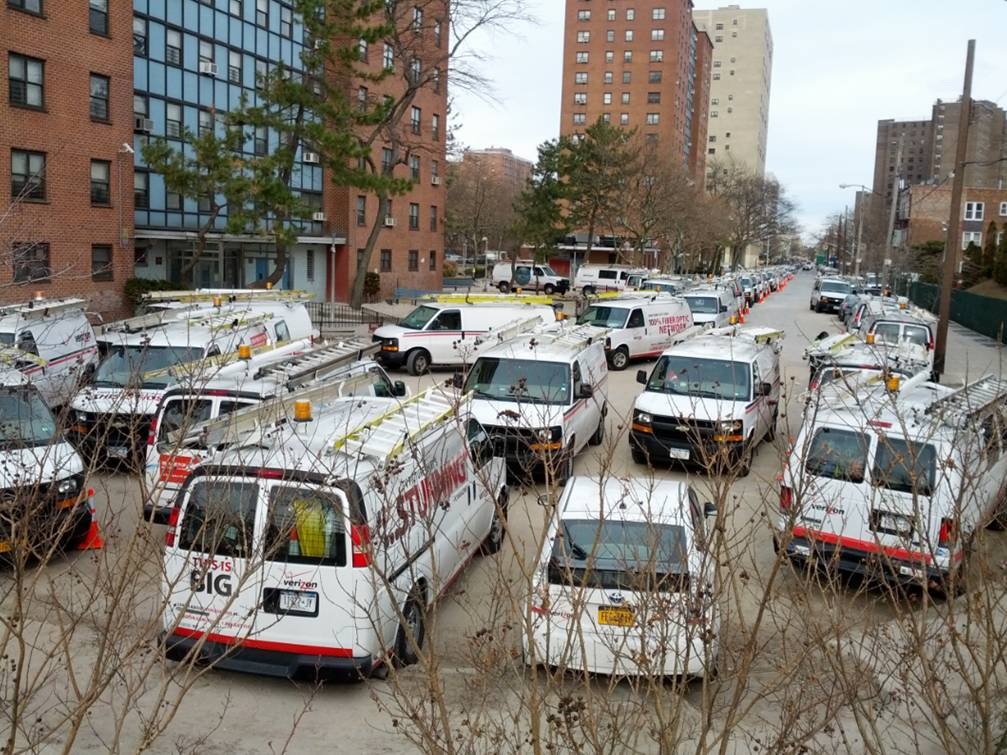This photograph captures a bustling urban scene on an overcast, fall or winter day. Taken from behind some bare bushes and trees, the image reveals a busy street lined with numerous maintenance vans, most likely belonging to Verizon, as indicated by the visible logos and text on a few of them. These white vehicles, some equipped with ladders, are situated in what appears to be a cul-de-sac. Orange cones are strategically placed along the street, suggesting a significant maintenance operation in progress. The backdrop features towering brick and glass buildings, likely high-rise apartments or office buildings, adding to the urban atmosphere. There are additional cars parked on the street, which may belong to employees or local residents. The overall scene is set under a cloudy sky, accentuating the cold, barren feel of the season.